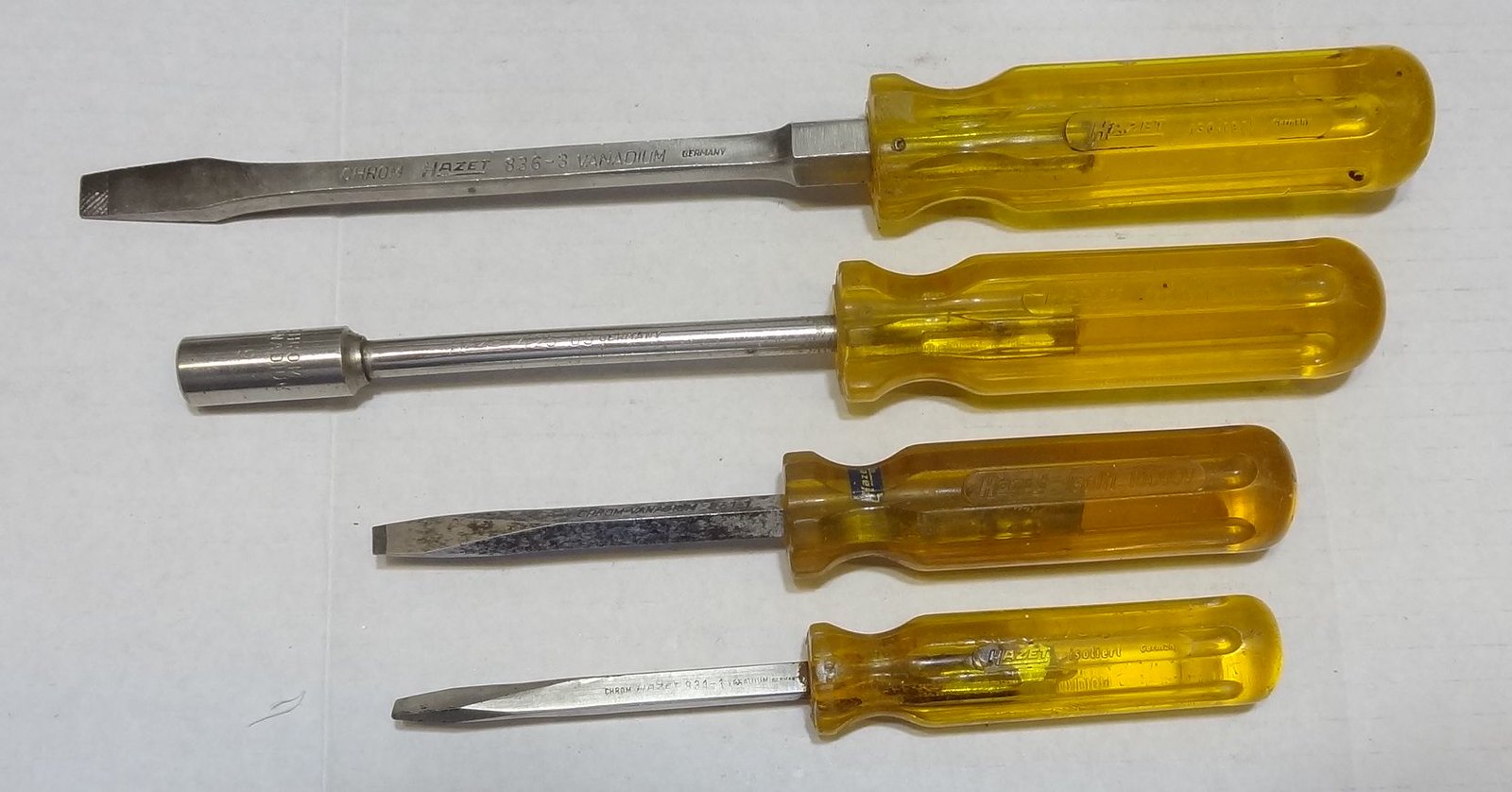This photograph features a central arrangement of four screwdrivers, all from the same manufacturer, HAZET 836-3 Vandium, as denoted by the etching on the metal part of each tool. Set against a smooth, light gray surface with faint lines and a small scratch resembling a hair in the left corner, the screwdrivers are meticulously organized from the largest at the top to the smallest at the bottom. Each tool boasts a yellowish-gold, transparent plastic handle positioned on the right side. 

The topmost tool is a long-handled flathead screwdriver, characterized by its transparent yellow handle and standard flat end. Below it is a slightly smaller tool with a similar handle but a blunt, cylindrical socket end. The third tool in the sequence is another flathead screwdriver, shorter than the previous two. Lastly, the smallest screwdriver, also with a yellow handle, features a textured flathead. Together, these four screwdrivers create a harmonious visual centered in the frame, emphasizing both their uniform make and varied sizes.